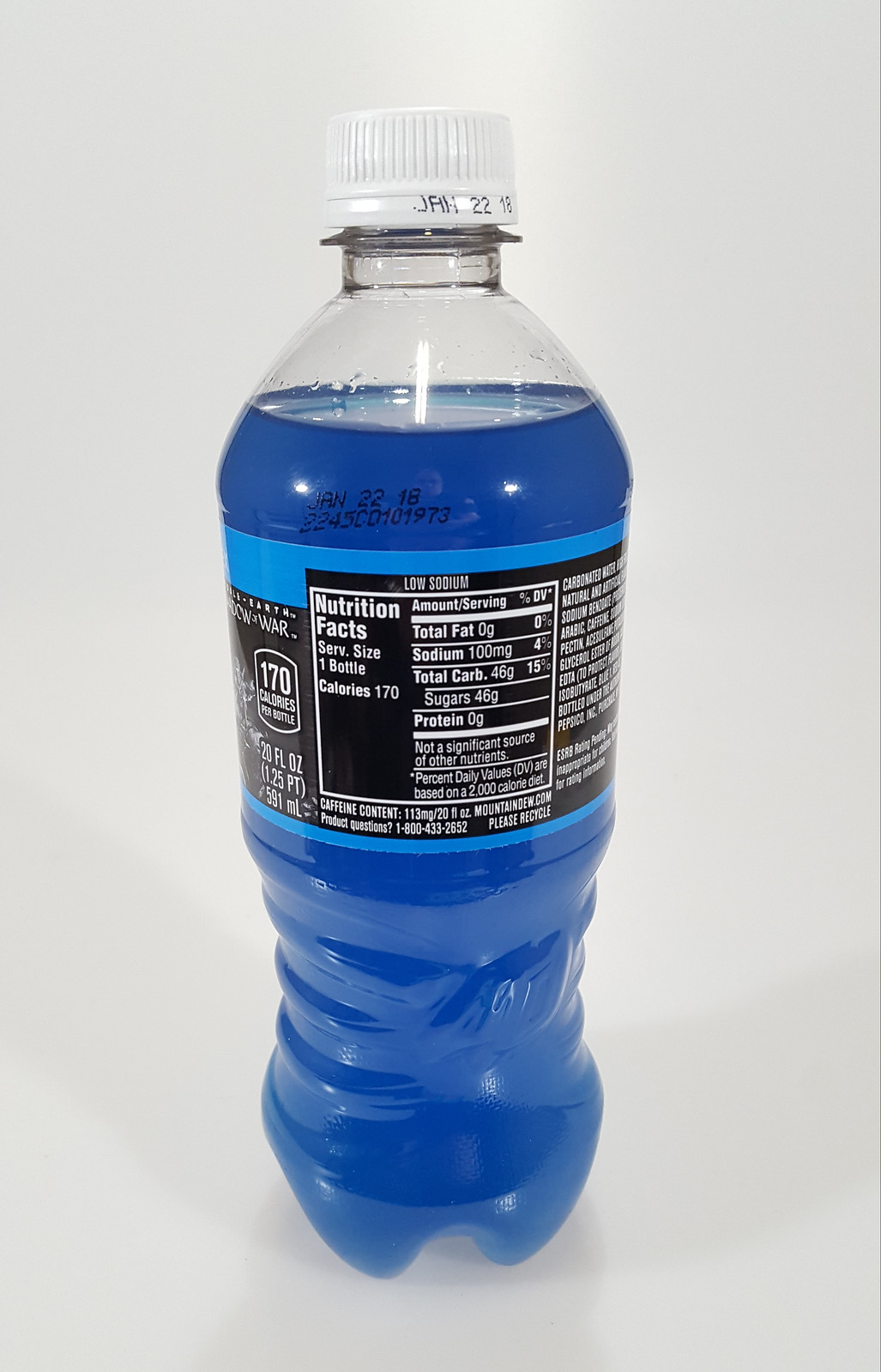This is an up-close photograph of a bottled drink, presented in a clear soda bottle. The drink is a deep blue color, and its label features a dark blue band at both the top and bottom, with a black background and white lettering in between. The brand name is not visible. The white cap and the side of the bottle indicate that the expiration date is January 22, 2018. Nutritional information displayed on the side of the bottle reveals that the drink contains 0 grams of fat, 100 milligrams of sodium, 46 grams of carbohydrates, 46 grams of sugar, and 0 grams of protein. Additionally, the top of the bottle reflects the image of the photographer, who appears to be a bald man wearing a short-sleeved black t-shirt.